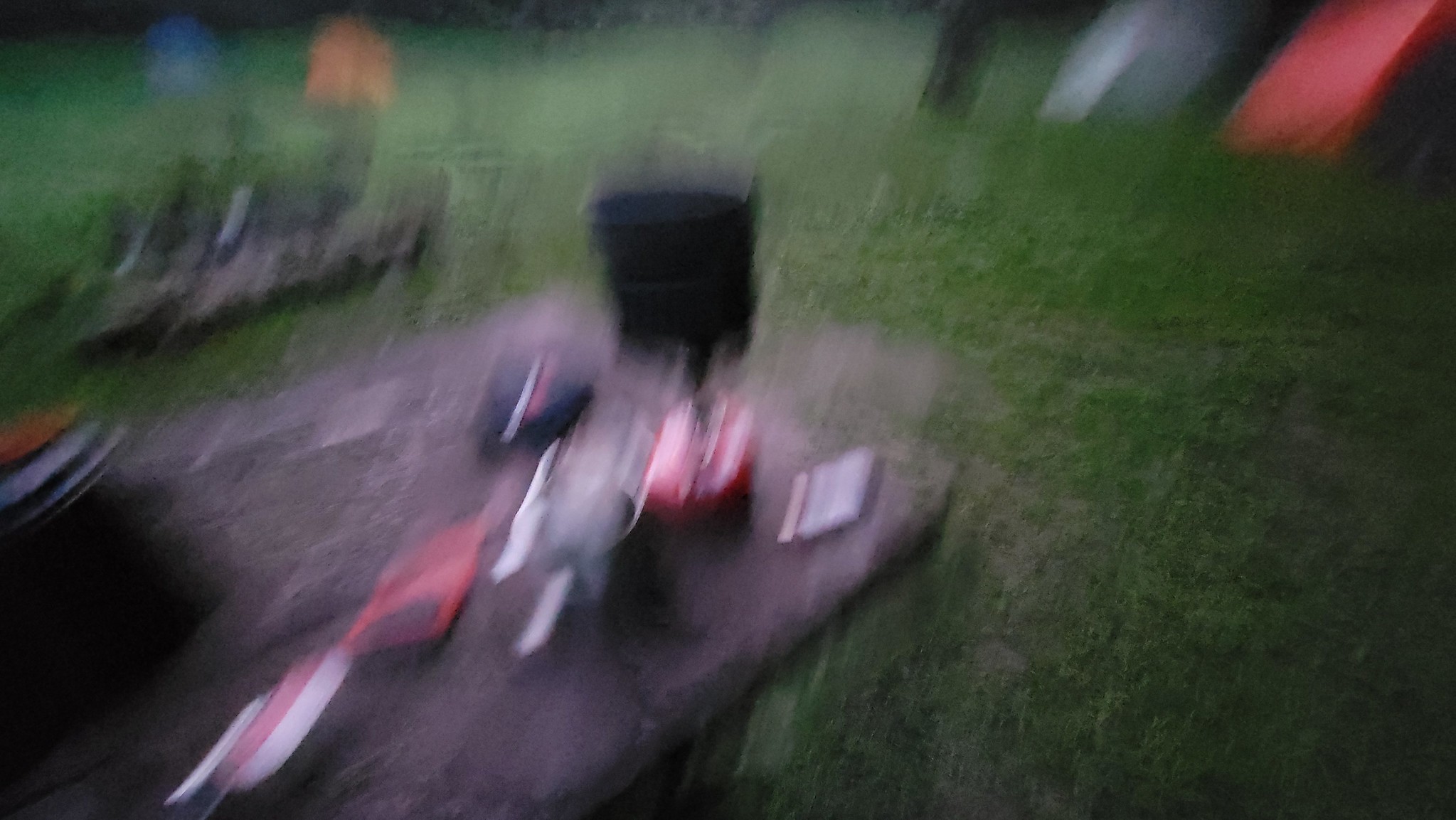The photograph is an outdoor, heavily blurred landscape image, likely due to camera motion when taken. The scene is dominated by dark green grass covering much of the area. In the foreground, there's an elevated structure resembling a table crafted from dark, bark-colored reclaimed wood with a noticeable join line running diagonally from the bottom left to the center of the frame. Atop the table, we can discern several indistinct items: a knocked-over plastic cup with a possible straw, a dark cylindrical object, and a few ambiguous items—one possibly being a train ticket or a tobacco packet.

Some blurred tools or objects are present, including a colander-like shape with an orange base and black parts, an orange tool bag potentially holding Allen wrenches, and a black bag with unclear red and white lettering. The background features a reddish object that might be a children's slide, a cylindrical black pot, and what seems to be a stone-lined fire pit encircled by green leaves and some silver elements. Off to the right, there appear to be a red and white tent or similar structure. The photograph, likely taken near evening, carries a palette of reds, oranges, blacks, and grays amid the greenery, adding to the scene's vague yet colorful composition.